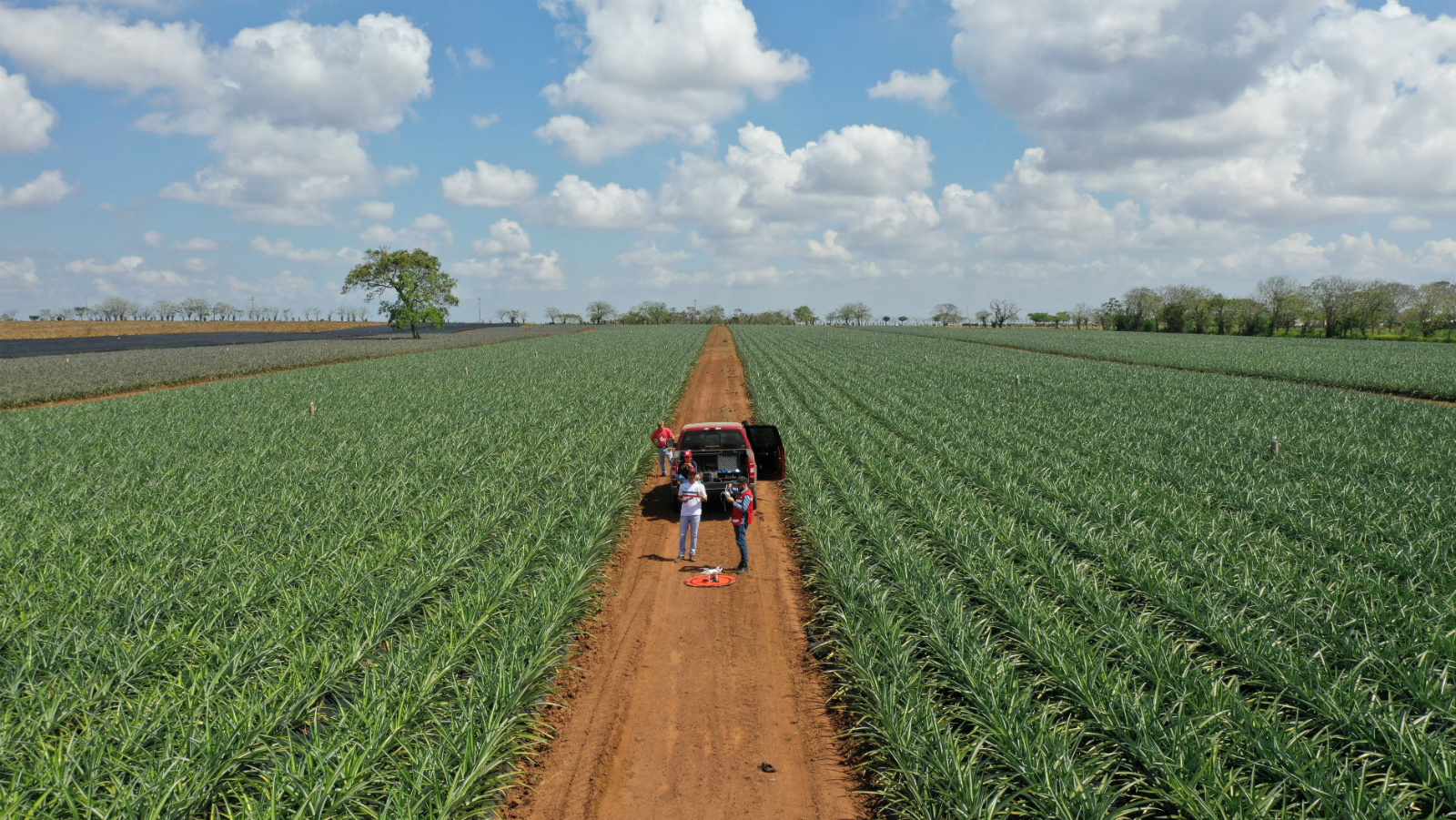This photograph depicts a vast farm field with a wide, horizontal expanse. Tall, green crops flanking a long dirt road stretch from the bottom center of the image into the distant background. In the middle of the scene, an SUV or pickup truck with its doors open is positioned on the dirt road. Surrounding the vehicle are four individuals: one wears blue jeans and a white shirt, another is dressed in blue jeans, a blue shirt, and a red vest. The remaining two figures are less discernible but are also gathered near the truck. The distant horizon showcases a mix of scattered trees to the right and left. Above, the sky forms a backdrop of blue interspersed with white and gray clouds, illuminated by the shining sun. There appears to be a sprinkler or another round object further in the distance, though details are indistinct. The scene suggests the group may be inspecting or tending to the crop in some manner.